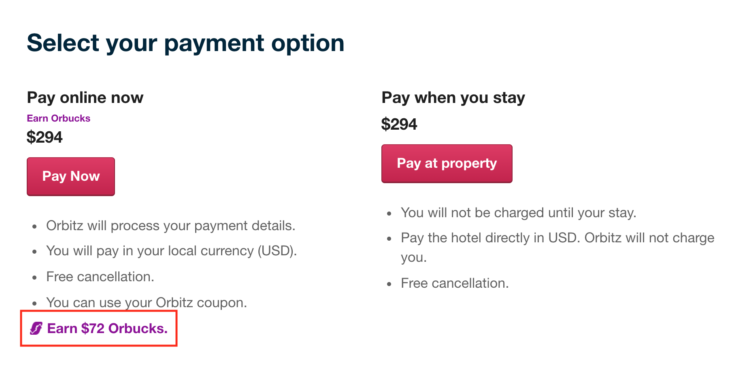The image is a rectangular web page section designed for selecting a payment option. At the top in large, bold black text, it reads, "Select Your Payment Option."

Two payment options are presented side by side:

1. **Pay Online Now for $294**:
   - Encased in a red box with white text that says, "Pay Now."
   - Below are bulleted points:
     - Orbitz will process your payment details.
     - You will pay in your local currency, USD.
     - Free cancellation.
     - You can use your Orbitz coupon.
   - Additionally, there is a red-outlined box featuring purple text that announces, "Earn $72 Orbucks."

2. **Pay When You Stay for $294**:
   - Encased in a red box with white text that says, "Pay at Property."
   - Below are bulleted points:
     - You will not be charged until your stay.
     - Pay the hotel directly in USD.
     - Orbitz will not charge you.
     - Free cancellation.